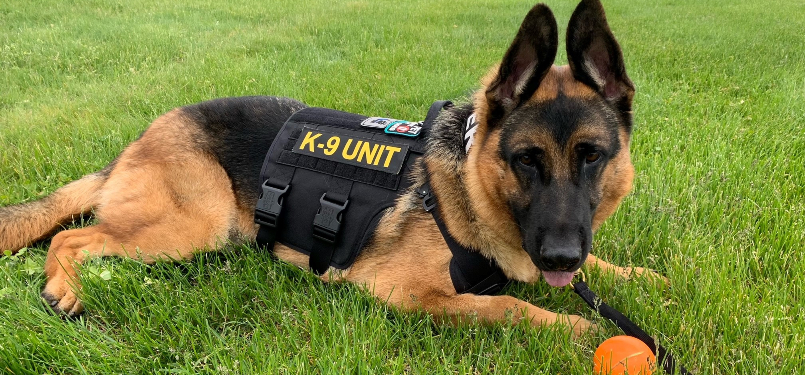In this meticulously detailed horizontal photograph, a German Shepherd lies on a well-manicured, bright green grass lawn, creating a peaceful yet dynamic outdoor setting. The dog is oriented from left to right, with its tail visible on the left side and its head lifted, mouth slightly open, revealing a gently panting tongue as if catching its breath. The German Shepherd exhibits the classic breed markings: a black face with long, somewhat drooping black ears, a tan body, and a distinctive black saddle design on its back. Clad in a black harness with bold yellow letters spelling "canine unit," along with some additional indistinguishable patches, the dog exudes an aura of training and purpose, likely linked to police or military roles. Additionally, a black leash connected to its collar extends near an orange tennis ball positioned just in front of the dog, hinting at recent playful activity. This well-fed and healthy canine looks directly towards the camera, capturing its alert and intelligent demeanor amidst the serene and inviting grassy backdrop.